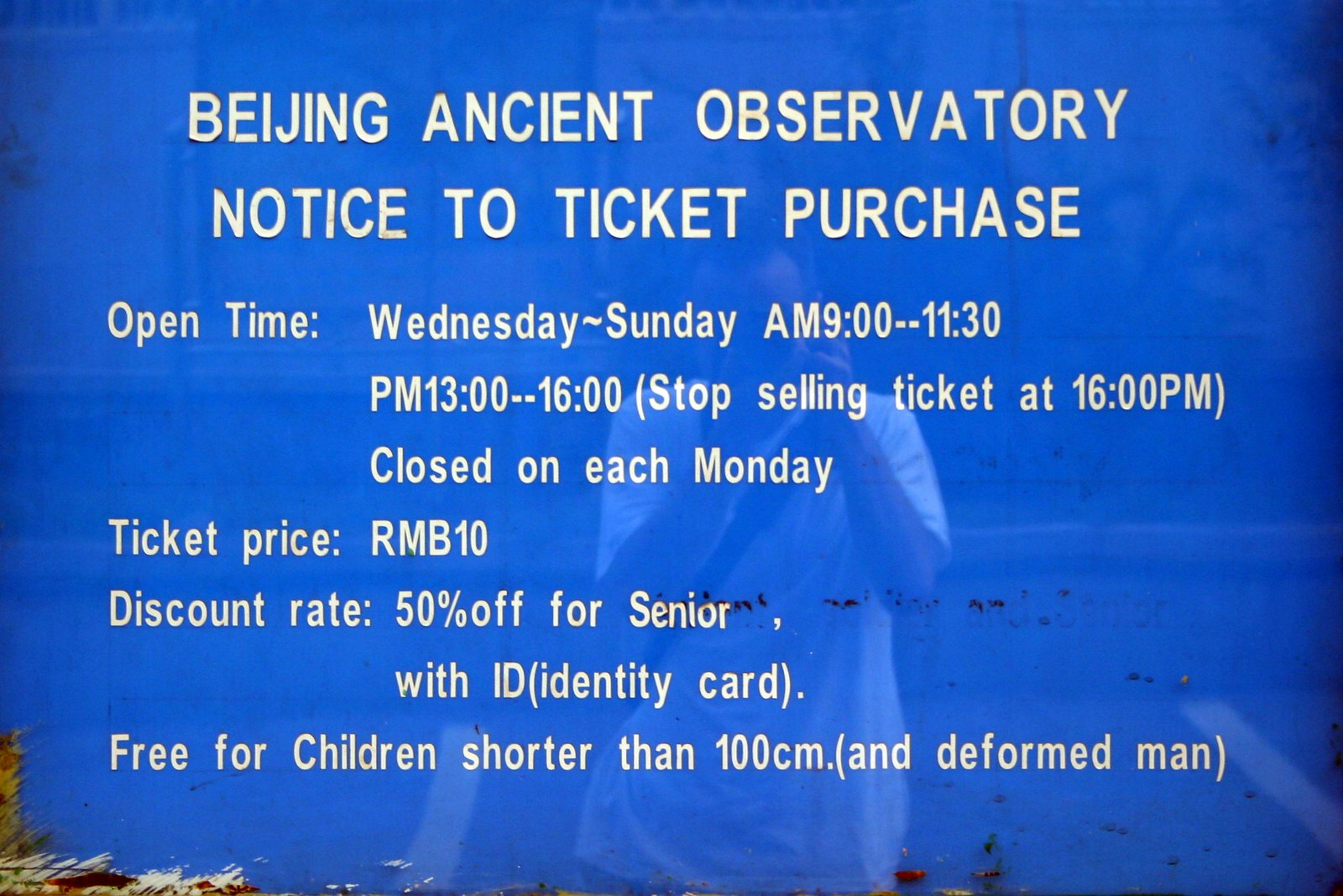The image is a metallic blue sign advertising the Beijing Ancient Observatory. It features a reflective surface, revealing someone in a white shirt taking a photo of the sign. The text on the sign, written in white font, provides detailed information on ticket purchasing. The observatory is open from Wednesday to Sunday, with hours from 9 a.m. to 11:30 a.m. and 1 p.m. to 4 p.m., with the last tickets sold at 4 p.m. It is closed every Monday. Ticket prices are listed as 10 RMB, with a 50% discount for seniors presenting an ID card. Additionally, children shorter than 100 centimeters and handicapped individuals are admitted for free.